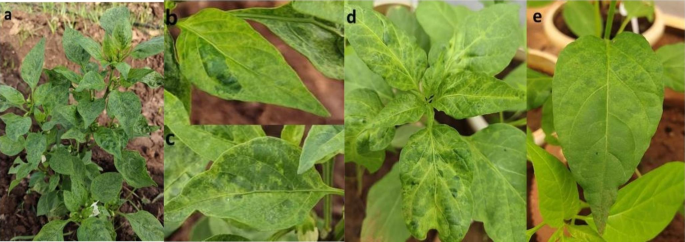The image consists of a single large rectangular photo compiled from five smaller individual photos, each labeled A, B, C, D, and E. Photo A displays a whole plant with green leaves situated against a dirt backdrop, resembling a potato plant. Photo B, located to the right of A, is a close-up image highlighting a spear-shaped leaf oriented to the right. Directly below B is Photo C, focusing on a rounder spear-shaped leaf facing to the left. Photo D, positioned to the right of B and C, offers an overhead view of the upper portion of the plant. Finally, Photo E, to the right of D, is another detailed close-up of a spear-shaped leaf, showcasing its intricate vein structure and oriented downward. Each photo together emphasizes different perspectives and details of the same or similar plant, focusing on the leaf shapes and orientation.